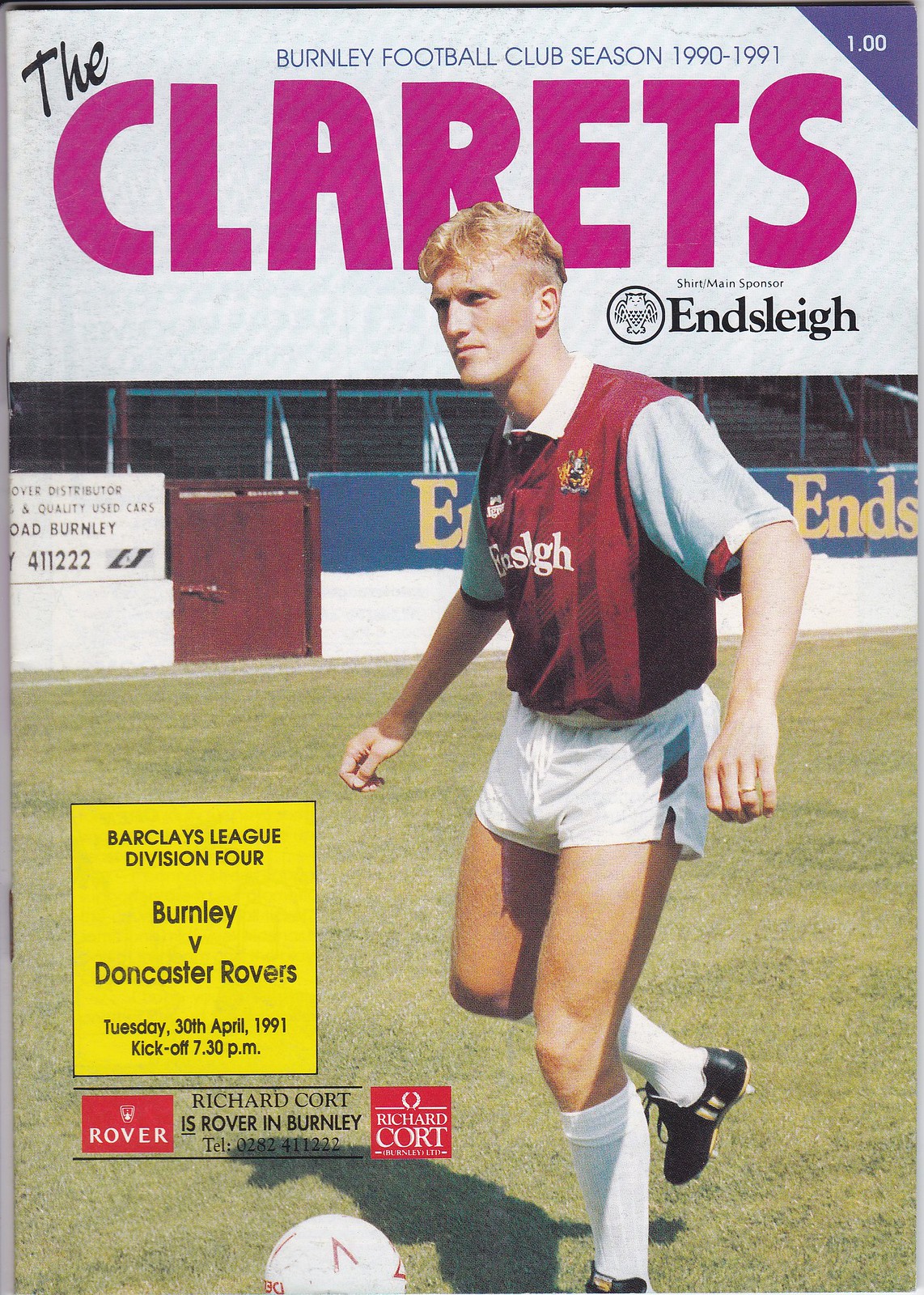The cover of the football program features a Burnley Football Club player prominently in the center. He wears a red jersey with light blue sleeves and "Enslay" as the sponsor written on the front, paired with short white shorts, white knee-high socks, and black cleats. Positioned in front of him is a soccer ball, suggesting he is about to kick it. At the top of the cover, the title "The Clarets" is displayed in large pink letters, with "Burnley Football Club, Season 1990-1991" written above it. Beneath "The Clarets," the sponsor "Enslay" is mentioned again, accompanied by its symbol to the left. The top right corner has a blue triangle displaying a price. Towards the bottom left, a yellow rectangle contains black text with details about the match: "Barclays League Division IV, Burnley vs. Doncaster Rovers, Tuesday, 30 April 1991, kickoff 7.30 p.m." To the right of this, there's a red box with "Rover" written in white font.